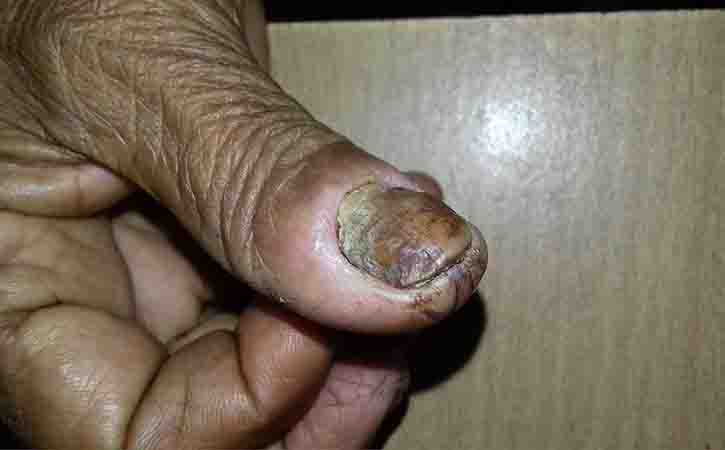The image depicts a disturbing close-up of a person's thumb afflicted with gangrene, prominently displaying the tip of the thumb and the area up to where it joins the hand. The thumbnail exhibits stark discoloration, with a brownish gray hue at the base transitioning to a brownish purple near the top. The skin on the thumb is visibly cracked with dark brown fissures, while the surrounding skin displays a mix of pink and purple tones, suggesting infection and possible swelling. The thumb, as well as the rest of the hand, appears wrinkled and dirty, which may indicate neglect or prolonged exposure to harsh conditions. The hand rests near the left side of the frame on a smooth, yellowish-brown wooden table, which reflects a bright light in the upper right area of the image, contrasting with the unsettling appearance of the infected thumb.